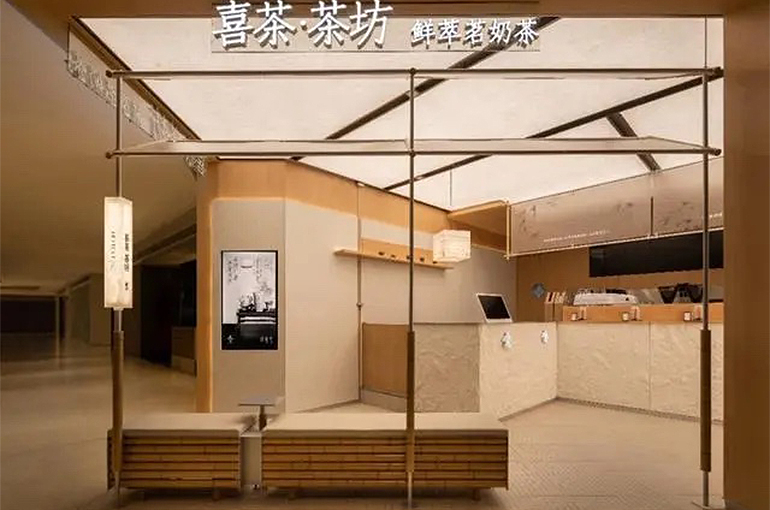This detailed illustration depicts the interior of a meticulously designed milk tea shop, situated within a shopping mall. The shop occupies a cozy corner, and an elegantly crafted banner, inscribed in Chinese characters, prominently announces it as a milk tea destination. The overall decor exudes warmth, achieved through the generous use of natural wood and bamboo across benches and ceilings. The scene is well-lit, enhancing the inviting ambiance of the shop. Although the background of the mall is shrouded in darkness with no lights, indicating an after-hours setting, the image captures the tea shop in vibrant clarity. No people are present, suggesting that this is a highly detailed 3D rendering, possibly created using SketchUp by an architect or a designer.